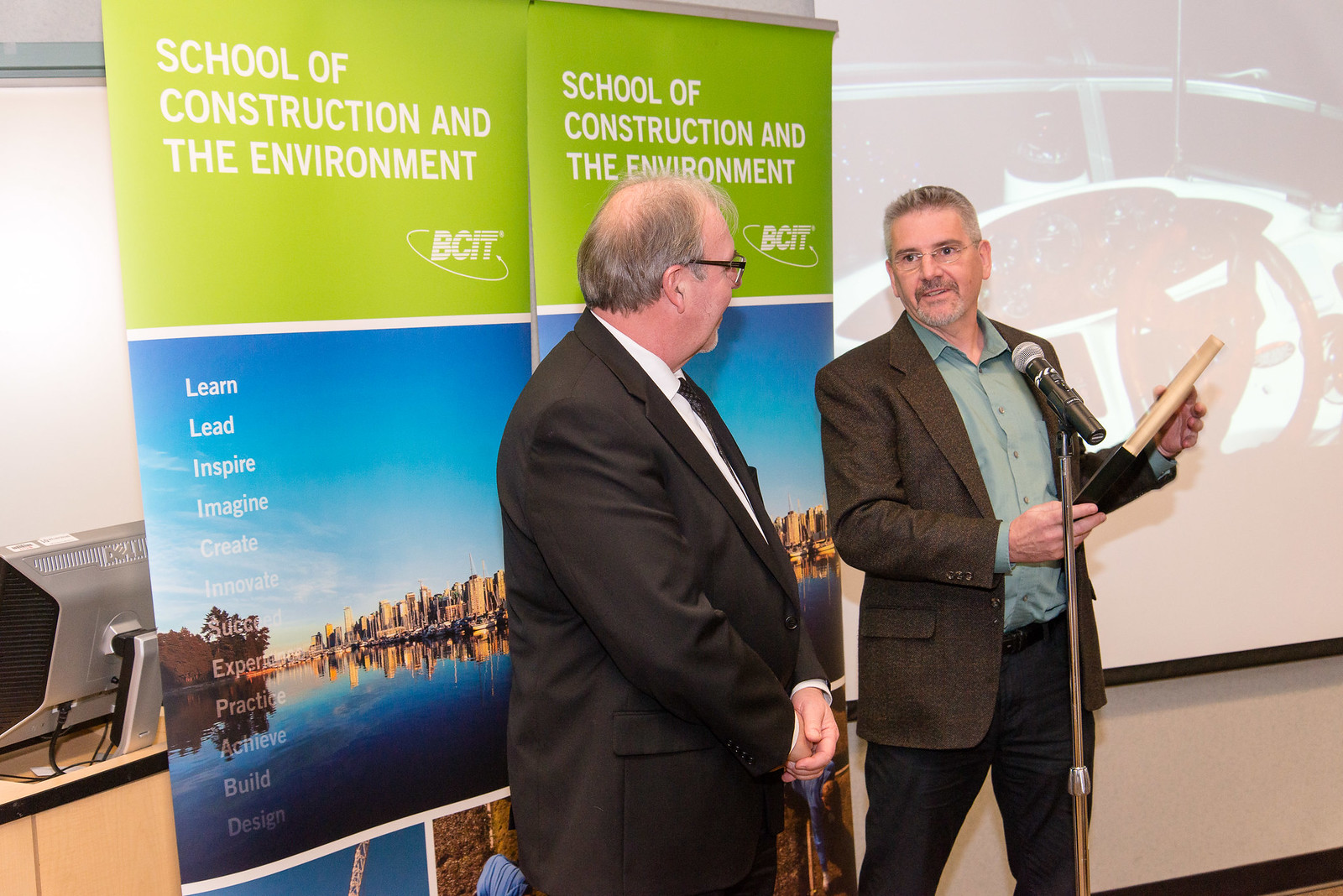In the photograph, two men are captured mid-presentation at a conference, standing behind a microphone. Both are dressed formally; the man on the left, who is slightly balding and heavyset, wears a black suit with a white button-down shirt and black tie, and sports glasses. His expression is directed towards the other man. The gentleman on the right has light-skinned, buzz-cut hair, and a mustache. He is clothed in a brown sport coat paired with a green shirt and dark pants, holding a book with both hands. Both men appear to be smiling and engaged with each other. Behind them is a prominent banner featuring a green section at the top and a mid-section with a cityscape overlooking water, predominantly in shades of blue. The sign bears white lettering that reads "School of Construction and the Environment," with additional text including "BCIT," "LEARN," "LEAD," "INSPIRE," and "IMAGINE." To their right, a white projector screen displays indistinct images. The setting suggests they are on a stage, adding a formal atmosphere to their presentation.